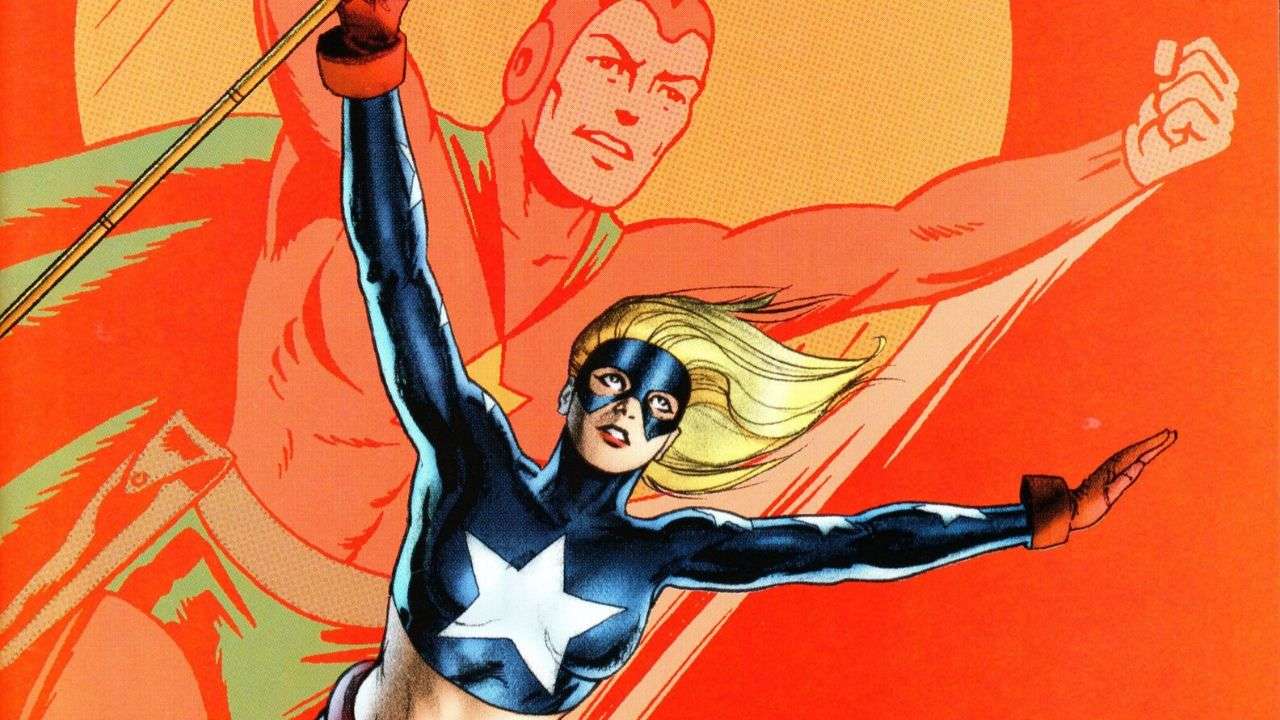The image is a vibrant horizontal comic book scene featuring two muscular superheroes flying toward the upper right-hand corner. In the foreground, a blonde woman with shoulder-length hair swept by the wind dons a blue bodysuit that reveals her midriff. Her striking outfit includes a white star on her chest, three white stars along each arm, red gloves with cuffs, and a Batman-like blue face mask. She holds a yellow rod in one outstretched arm. In the background, a much larger male superhero, painted in silhouette style, wears a long-sleeved orange crop top with red tights stretching over his head and cylindrical pieces covering his ears. He also sports a green underwear piece and a green cape with a red underside, flying with arms outstretched through red and pink streaks signifying speed and wind. There’s a large orange background, accentuated by a yellowish circle directly behind the male hero. The overall image is a detailed, close-up comic book artwork capturing a dynamic moment of two heroic figures in flight.